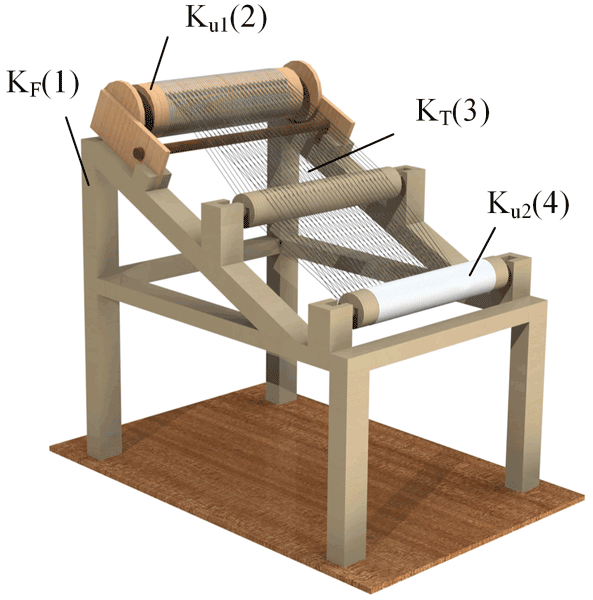The image depicts a detailed diagram of a non-electric, wooden weaving machine, likely a loom, set on a plain wooden board. This beige contraption features three progressively smaller rollers, with the largest roller positioned at the top, followed by a central roller, and the smallest roller at the bottom. Black strings run horizontally across the three rollers. Various parts of the machine are labeled with letters and numbers: the base is labeled "KF (1)," the top roller is identified as "KUL (2)," the central section with thin wires is marked "KT (3)," and the bottom roller, which appears to be wrapped in white paper, is labeled "KU2 (4)." The overall presentation suggests that the image is from a textbook or scientific reference, given the precision and annotation used to describe the machine's components.